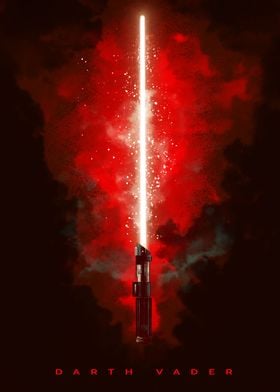This is a detailed poster connected to the Star Wars franchise, focusing exclusively on Darth Vader. The background is predominantly black, gradually shifting around the center into a dark, fiery red reminiscent of flames or smoke. In the middle of the poster, a lightsaber stands vertically, extending nearly from the bottom to the top. The lightsaber's handle is a sleek, high-tech design with a black grip, accented by gold bands and a slanted black piece near the top. A white-hot beam of light, surrounded by a red glow, emanates from the handle, scattering white sparkles and flecks around it. The red glow is so intense that it appears to generate red smoke or flames. Teal smoke is faintly visible near the handle. At the bottom of the poster, "Darth Vader" is written in widely spaced red letters, grounding the composition. This promotional image emphasizes the powerful and ominous presence of Darth Vader through its striking use of color and light.